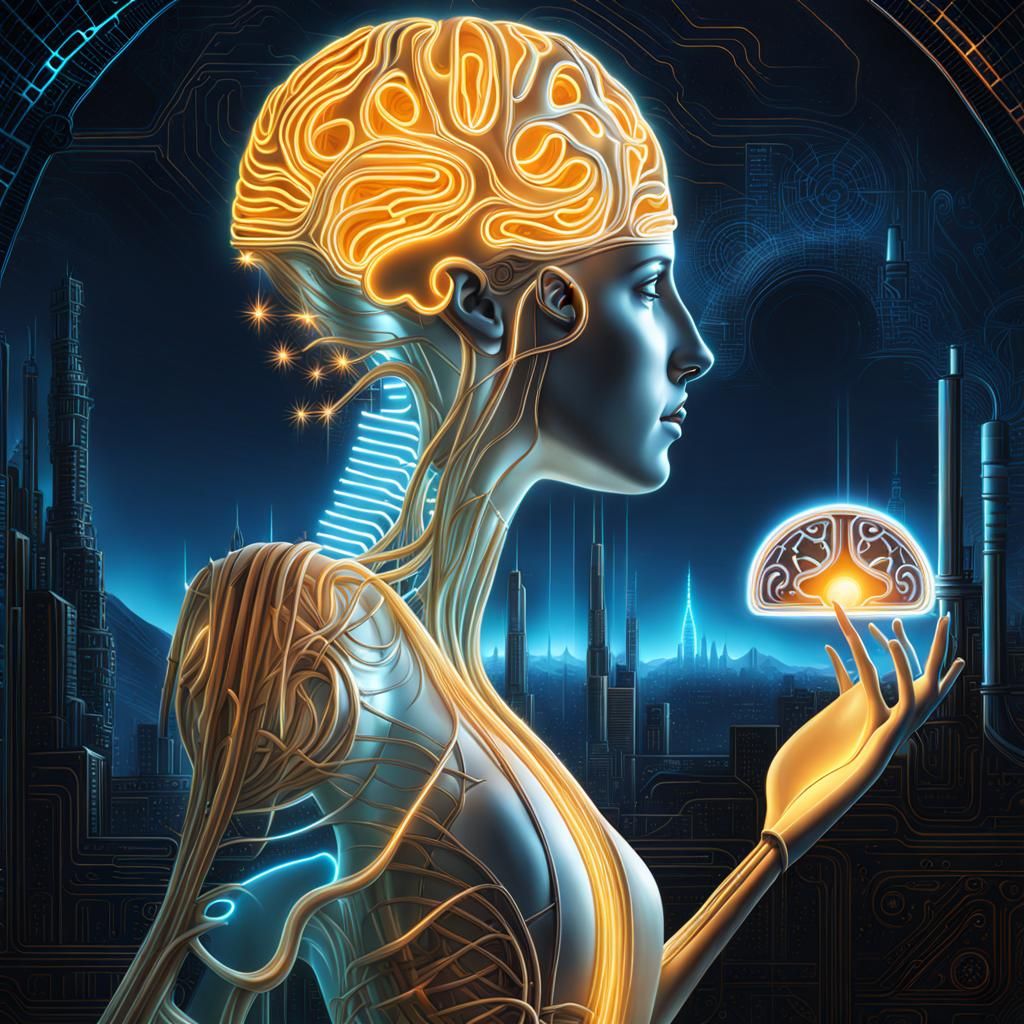The image presents a detailed and futuristic portrayal of a female robot in a side profile view, emphasizing her right side. The woman looks robotic, with a silvery grey complexion and visible mechanical features. Her brain, glowing with orange light, is exposed, revealing a network of orange lines and wires that extend throughout her body. These wires penetrate her neck, shoulders, and upper torso, giving her a highly cybernetic appearance. Notably, her left hand is outstretched and unusually adorned with seven fingers. 

Her body exhibits a light blue glow, particularly accentuating her spine with neon blue hues. The entire figure has a semi-transparent quality, making internal wiring and structural elements visible, which look like veins. The image is set against a backdrop of dark, futuristic skyscrapers illuminated by moonlight and interspersed with blue glows, contributing to the industrial and advanced atmosphere. Tall buildings dominate the background with intricate blue lighting, enhancing the high-tech and intricate setting of this vividly clear and dynamic artwork.